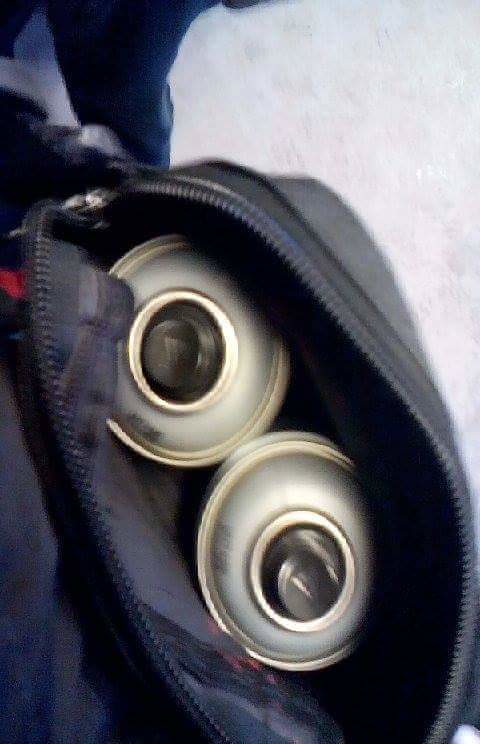The image is a blurry photograph of the inside of a partially unzipped navy blue, almost black fanny pack or carryall bag. Inside the bag are two upright aerosol cans, each with a silver body and a black top. The bag features a plastic navy blue zipper, and the background reveals a white floor. In the background, there appear to be two legs clad in black workout pants or tights, suggesting the presence of a person. The purpose of these aerosol cans is not certain, but they could potentially be used by a street artist or muralist, given the typical use of such items for spray painting. The image is somewhat unfocused, making it difficult to discern additional details.